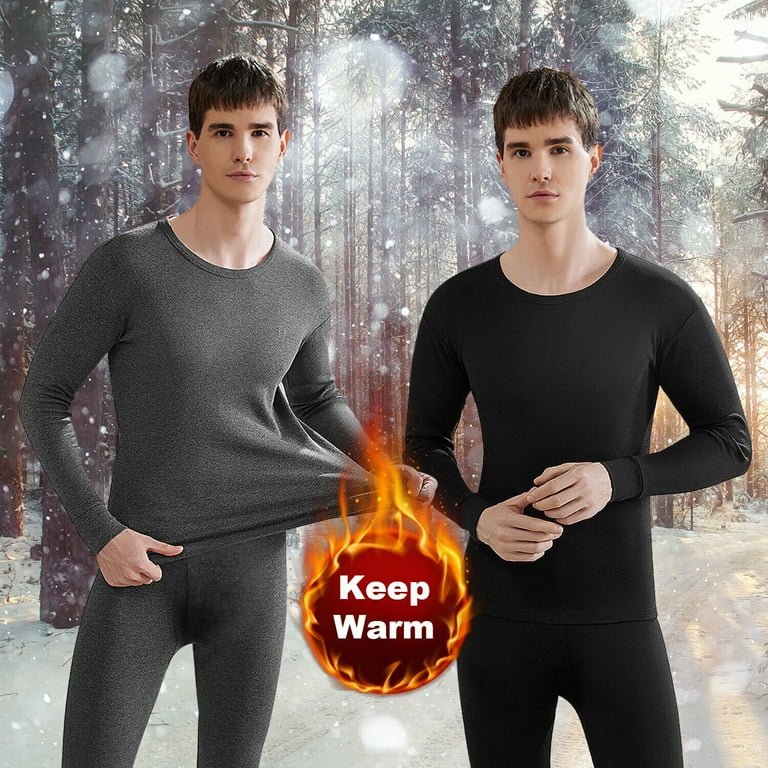This square image, likely styled as a clothing advertisement, prominently features either a pair of twins or the same young man photographed and composited together against a scenic winter backdrop. The background showcases a serene wooded area with tall, slender pine trees blanketed by falling snowflakes, emphasizing a wintery atmosphere with snow covering the ground.

In the foreground, centrally placed at the lower part of the image, a fiery red circle adorned with orangish-yellow flames arcs upwards from the top, lending a vibrant and warm contrast to the wintry scene. Within this circle, bold white letters spell out the phrase "KEEP WARM," underscoring the advertisement’s message.

On the left side, the young man is dressed in a gray, round-neck, long-sleeved thermal shirt. With his right hand, he grips the hem of the shirt at his hip, while his left hand stretches the fabric outward towards the "KEEP WARM" logo, suggesting the shirt’s flexibility and comfort. On the right side, the same young man—or his twin—is clad in a similar form-fitting thermal outfit, the snug fit clearly highlighting the garment's contours. His hands are clasped together at his waist, elbows slightly extended, subtly showcasing the well-fitted nature of the thermal wear.

Both young men, or twins, are Caucasian with dark brown hair, further adding to the cohesive visual appeal of the advertisement. The contrasting elements of fire and snow within the image effectively highlight the thermal clothing's warmth and comfort, even in the coldest conditions.